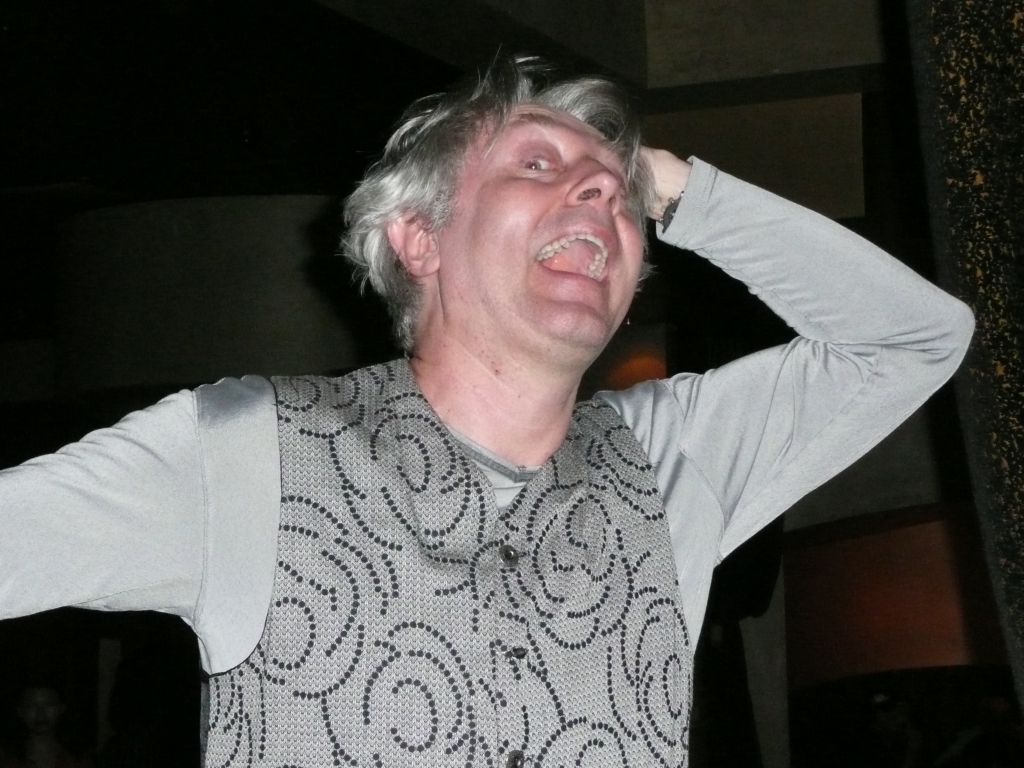The image depicts an older Caucasian man with short gray or silver hair, and a clean-shaven face marked with subtle wrinkles. He's wearing a gray patterned vest over a metallic, long-sleeved gray undershirt. His posture is dynamic; his head is slightly leaned to the left, eyes fixed directly on the camera, while his mouth is half-open in a surprising, somewhat wild smile. His left arm is cocked and bent behind his head, and his right arm extends outward, though only the shoulder and a hint of the arm are visible. The brightly lit man stands out sharply against the dark background, suggesting the photo was taken either at night or in a poorly lit indoor area with a flash. Behind him, there is a speckled concrete wall on his right and what appears to be a concrete stairway or platforms. In the lower left corner, the vague silhouette of another person, resembling a mannequin, can be seen. The image captures from about the third button of his vest upwards, with no view of his hips or legs. The overall scene is captured in a moment of spontaneous animation and contrasting lighting.